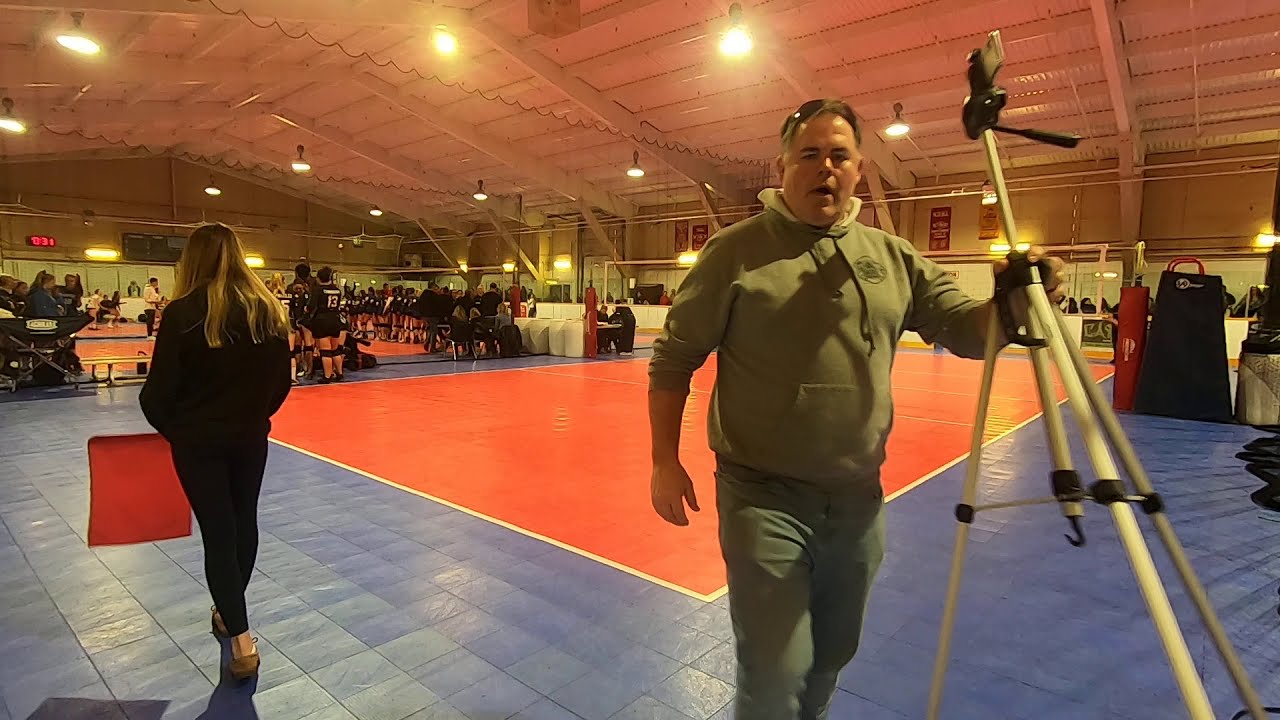This image captures the inside of a brightly lit gymnasium, featuring a distinctive floor layout where a large red square mat is bordered by blue square tiles. In the foreground, an older gentleman, dressed in beige attire with sunglasses propped on his head, holds a tripod with a camera attached. To his left, a woman with blonde hair, clad in black clothing and brown shoes, is seen walking away, holding a red flag. The background reveals an array of athletes or individuals standing around, wearing black jerseys with numbers, indicative of some sporting event. Notably, above the woman's left shoulder, a man in a white outfit, likely an official or judge, is observed overseeing the scene.